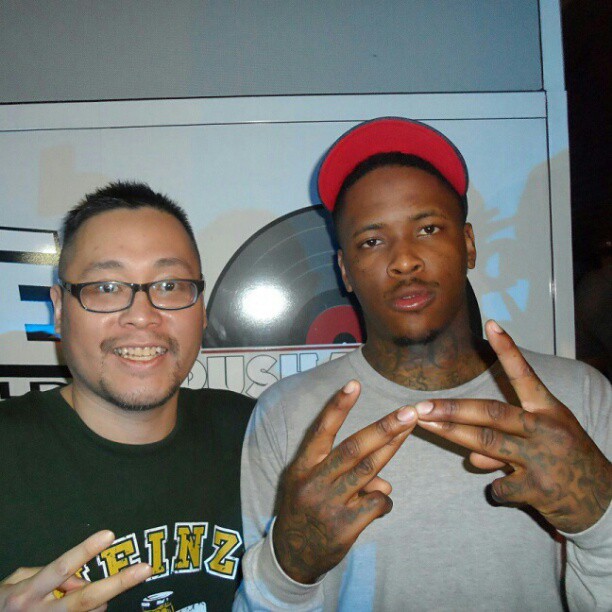The photograph captures two men standing side by side, likely at a meet-and-greet event in front of a backdrop featuring icons for a specific company or music publisher. The man on the right, presumed to be a musician, is an African American with very dark brown skin and short black hair. He wears a red baseball cap with a red underside on the bill and a long-sleeve, heather gray t-shirt. His tattoos are prominently displayed on his fingers, hands, and partly visible on his chest and neck. He stands with a serious demeanor, posing with a distinctive hand gesture recognizable to his fans. 

On the left stands an excited fan, possibly Hispanic, with tan-colored skin and very short, spiky black hair. He sports a black t-shirt with the word "Heinz" printed on it, and he flashes a peace sign with his hand. A slight mustache and goatee complete his look. The backdrop behind them includes a large record icon, contributing to the musical atmosphere of the event.